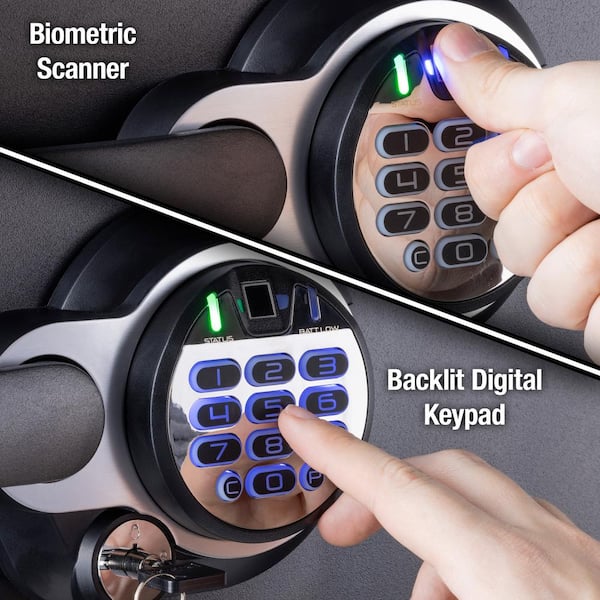The image is an advertisement guide for a safe featuring a biometric scanner and a backlit digital keypad. The image is divided into two sections. 

The top section, titled "Biometric Scanner," depicts a person with light skin placing their thumb on an electronic lock's fingerprint scanner. The scanner is equipped with a green status light and a blue battery low light. 

The bottom section, labeled "Backlit Digital Keypad," fully displays a keypad consisting of numbers 0 through 9, a 'C' button, and a 'P' button. The keypad is backlit with a blue hue, enhancing visibility. This part of the image also includes a depiction of a person entering a code, highlighting the presence of a turnkey mechanism for additional access. The safe itself is a blackish-gray color with lighter gray-silver accents around the handle.